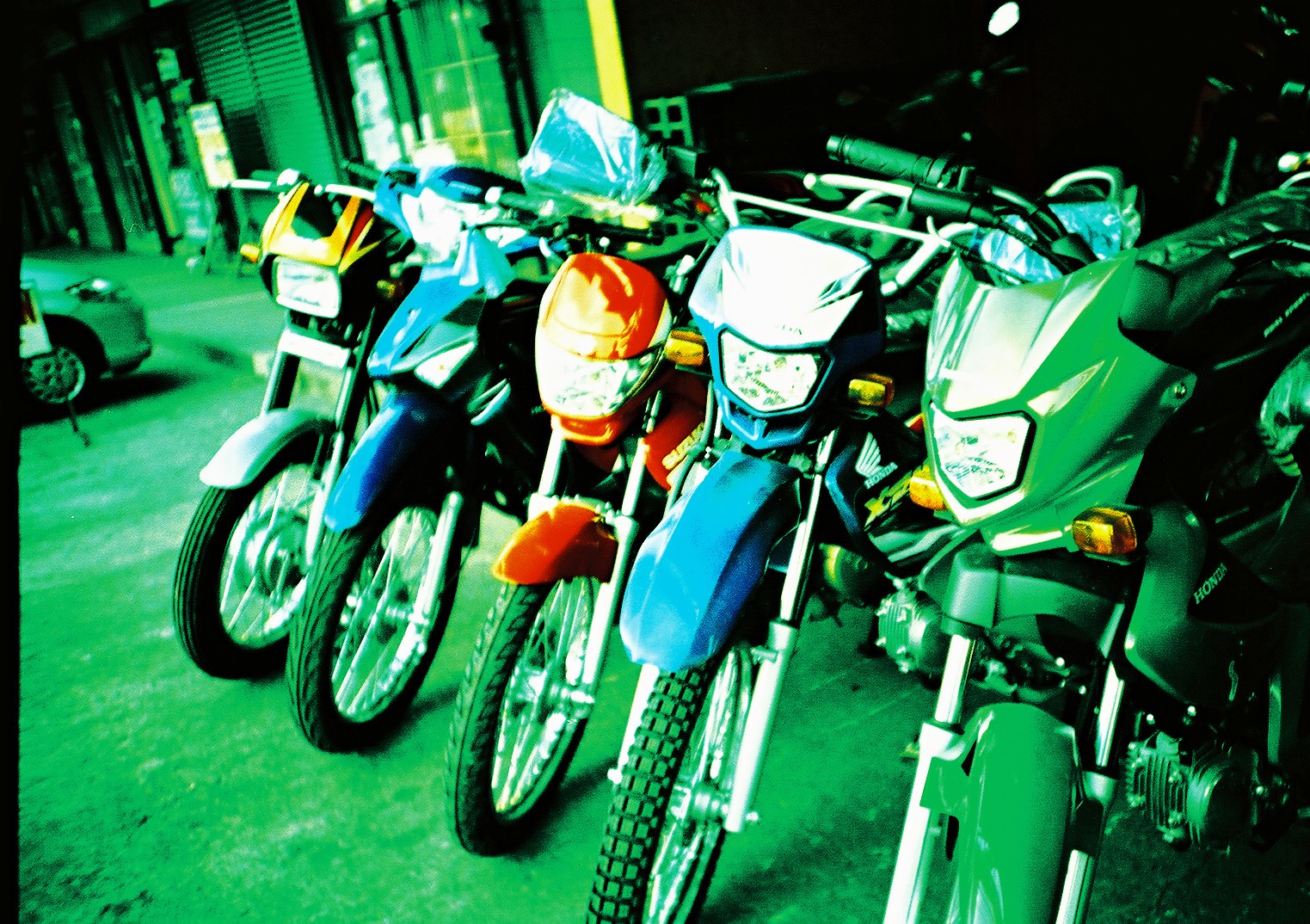The image depicts a lineup of five motorcycles parked in front of a storefront, with a portion of a car visible on the left. The photograph has a greenish tint, affecting the overall lighting and giving the background, which includes a garage or street scene, a distinct green hue. The motorcycles are arranged from left to right in the following color sequence: yellow, blue, red, blue, and green. Each bike has its headlights prominently centered, and various details such as fenders and handlebars are clearly visible. The scene is bathed in harsh light that emphasizes the vibrant colors of the motorcycles, making them stand out against the tinted backdrop.